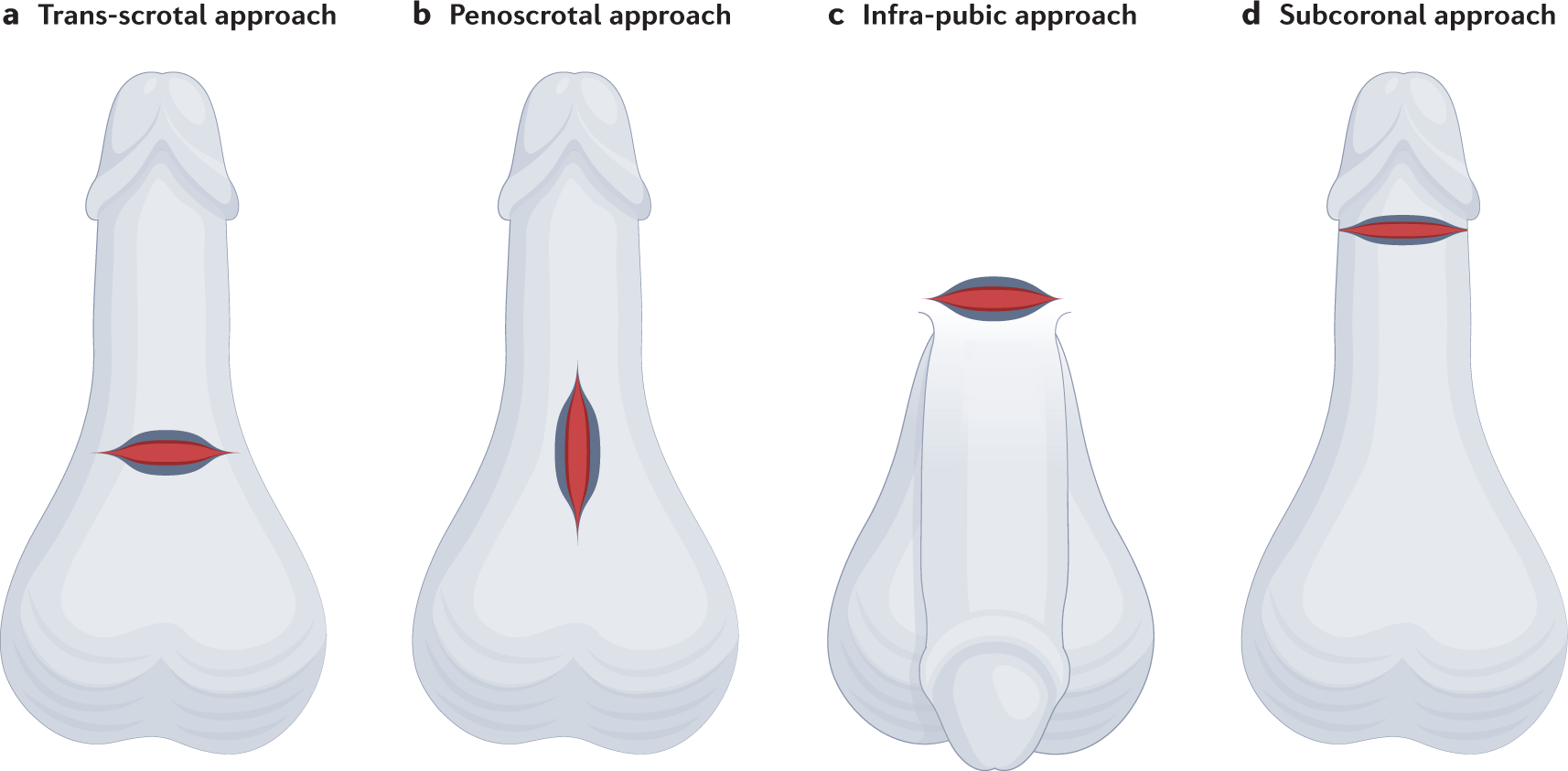The image appears to be an excerpt from a medical textbook, featuring four schematic drawings of a penis and testicles aligned in a row from left to right, labeled A through D. Each drawing illustrates different surgical approaches with corresponding incision sites. 

- **Drawing A** is labeled "Transscrotal Approach," depicting a penis pointed straight up with testicles at the bottom. There is a horizontal incision made between the testicular sac and the base of the penis.
- **Drawing B** is labeled "Penoscrotal Approach," showing the same orientation with the penis pointing up and the testicles below. This drawing features a vertical incision at the base of the penis, directly above the testicles.
- **Drawing C** is labeled "Infrapubic Approach," where the penis is oriented differently, pointing straight down with the testicles behind the shaft. The illustration shows a horizontal incision at the base of the penis, situated at the top of the drawing.
- **Drawing D** is labeled "Subcoronal Approach," returning to the same orientation as A and B, with the penis pointing up and the testicles at the bottom. A horizontal incision is placed just below the head of the penis.

All drawings are rendered in grayscale, set against a white background, and appear designed to illustrate the various surgical incision techniques for educational purposes.